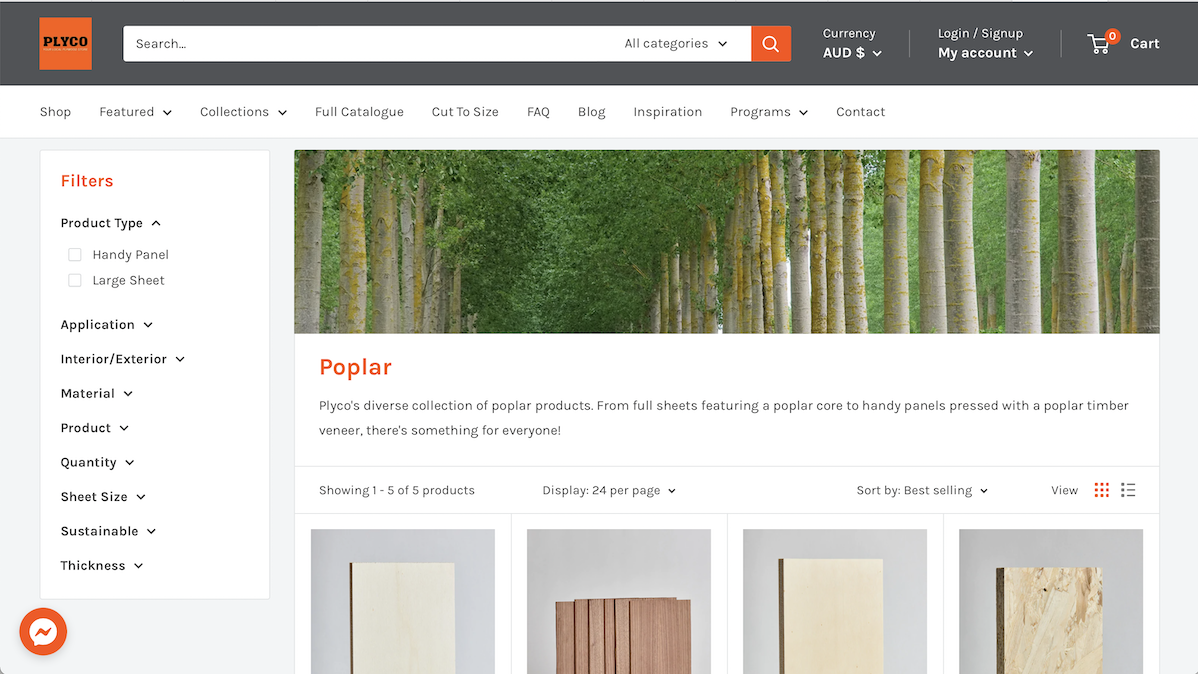This screenshot showcases the homepage of a website named Plyco. 

At the very top, there's a light gray bar housing various elements. The leftmost section features the Plyco logo, which is an orange square with black text. Adjacent to this logo is a search bar with a button at its right, displaying an orange square with a white magnifying glass icon. Following the search bar, there's a currency selection option denoted as AUD (Australian Dollar) with a dropdown menu for other currencies. Further to the right, there are links for logging in, signing up, and accessing "My Account." Near the top right corner, a shopping cart icon with a zero inside an orange circle indicates the cart status.

Beneath this gray bar lies a white horizontal navigation bar containing categories labeled: Shop, Featured Collections, Full Catalog, Cut to Size, FAQ, Blog, Inspiration, Programs, and Contact.

On the left side of the page, a vertical menu titled "Filters" is visible. This menu includes various dropdown options such as Product Type, Handy Panel, Large Sheet, Application (Interior, Exterior), Material, Product Quantity, Sheet Size, Sustainable, and Thickness. Currently, all dropdowns are closed except for one unnamed dropdown.

Visible in the bottom left corner is a distinct speech bubble icon with a lightning bolt through it, likely representing a chat or feedback feature.

The main content area features a prominent hero image, displaying what appears to be rows of trees, which may resemble bamboo. Overlaid text reads: "Poplar - Plyco's diverse collection of poplar products, from full sheets featuring a poplar core to handy panels pressed with poplar timber veneer. There's something for everyone."

Below this description, four inset photos display small strips of wood, representing a selection of products. Accompanying these images, options allow users to view one of five product types, display 24 items per page, sort by best selling, and toggle between different photo grid views.

This detailed depiction provides a comprehensive understanding of Plyco's website layout and available features on the homepage.